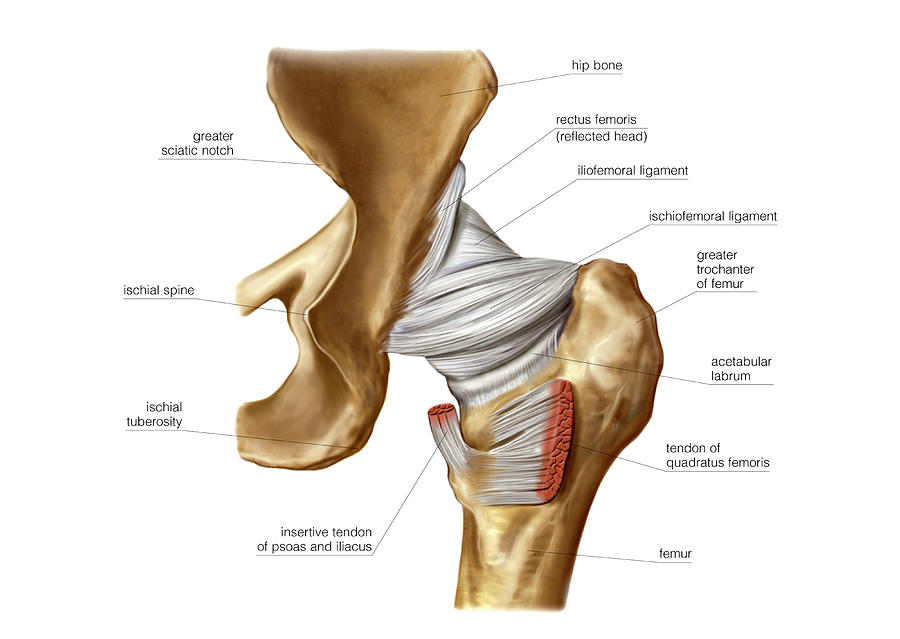This is a detailed medical textbook-style illustration depicting the anatomy of the hip bone and the proximal femur. The bones are rendered in light brown or tan hues, while the muscles and ligaments are illustrated in a whitish-gray, accentuated with red edges where the musculature is cut away. The background of the image is white, making the anatomical structures stand out clearly. The illustration features numerous labels with thin lines extending from the specific anatomical sections to horizontal lines above which the text labels are displayed.

Key labeled structures include:
- Hip Bone
- Greater Sciatic Notch, a notch in the hip bone
- Ischial Spine, part of the hip bone
- Ischial Tuberosity, a protrusion at the bottom of the hip bone
- Rectus Femoris (Reflected Head), a muscle
- Iliofemoral Ligament
- Ischiofemoral Ligament
- Greater Trochanter of Femur, a prominent part of the top of the femur
- Acetabular Labrum, a type of ligament/musculature at the top of the femur
- Insertive Tendon of Psoas and Iliacus, tendons near the hip area

All labels are in black text, with each label pointing to its corresponding part using fine lines. This detailed diagram provides a comprehensive view of the anatomical connections and structures of the hip region, ideal for educational purposes.